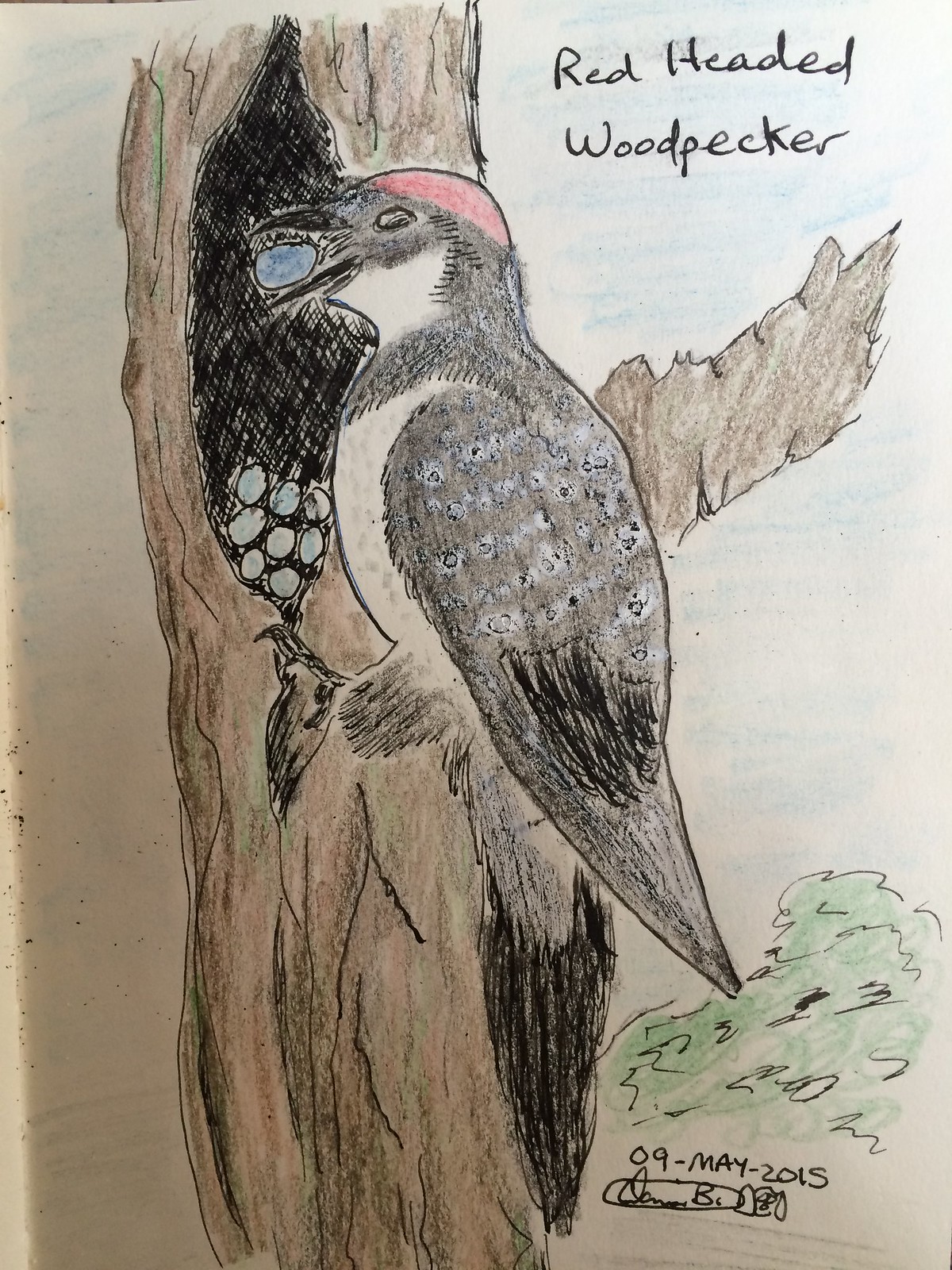This artwork, titled "99-2015," features a dynamic and detailed landscape. The sky, depicted in a serene blue hue, contrasts with the earthy brown tones of the ground. Scattered around the scene are dotted colored pencils and hints of ink, adding texture and depth. In the bottom right corner, the outlines of a bush are meticulously rendered in ink, with green leaves sprouting vibrantly. Dominating the center of the composition is a towering tree with rugged brown bark. Within a hollow of the tree, white objects resembling eggs or pebbles can be seen. Perched at the entrance of the hollow is a bird with a striking appearance: a red head, black wings, white body, and red temples, accompanied by black-tipped sides, a white neck, and a white chest. The bird's claws grip firmly onto the edge of the hollow, adding a sense of tension and realism to the artwork.